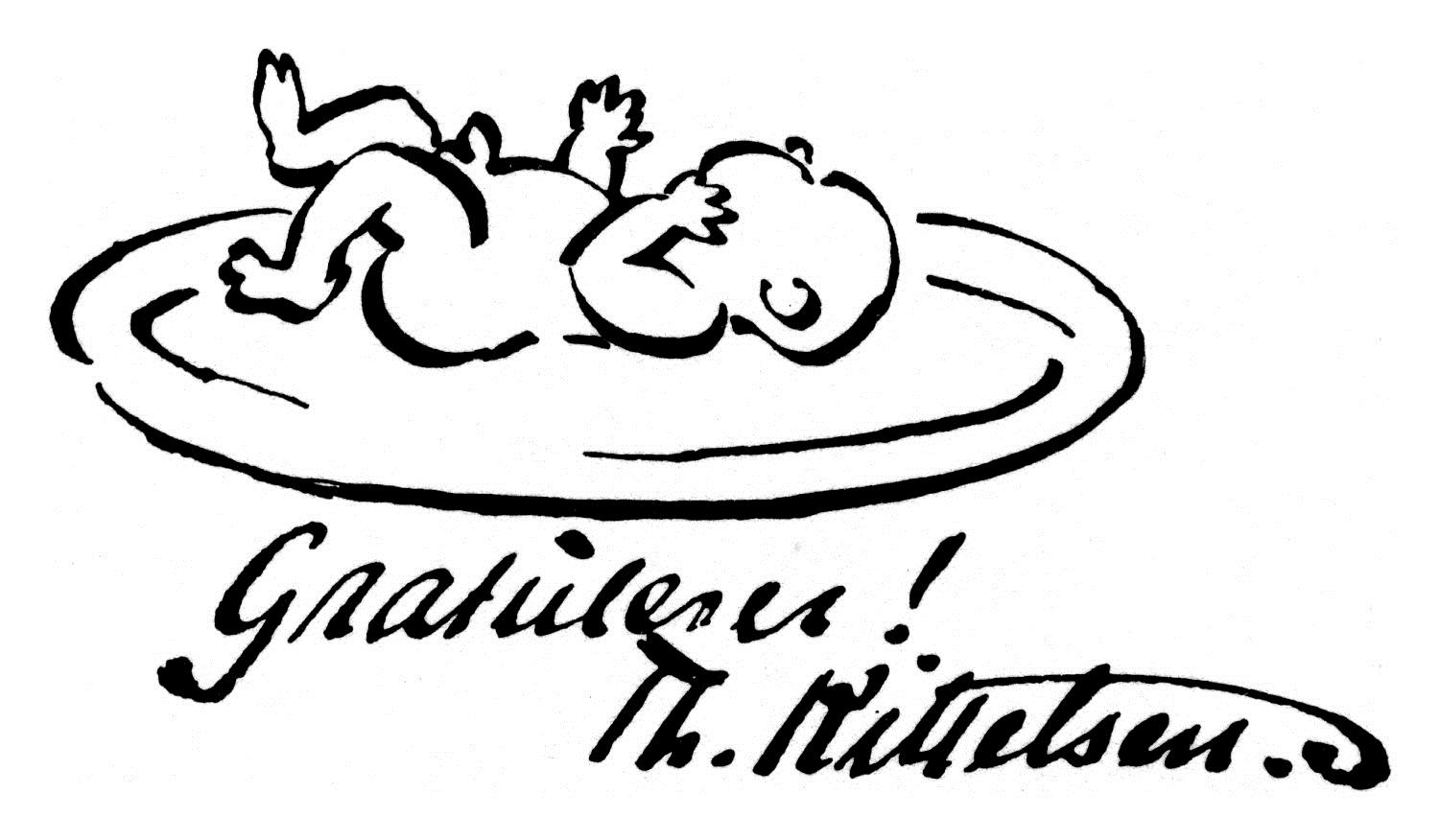This black-and-white drawing features a naked baby boy lying on his back with his head turned to the side, hands near his face, and legs stretched out. The baby appears to be resting on a round, oval object adorned with lines, which could represent a plate, a blanket, or a rug. Surrounding the baby, a cursive inscription in another language can be seen at the bottom, partially decipherable as "gratitudes" or a similar word, possibly congratulating a couple on their new baby. The drawing is simple yet detailed, and despite its monochromatic palette, it effectively highlights the baby as the central focus.